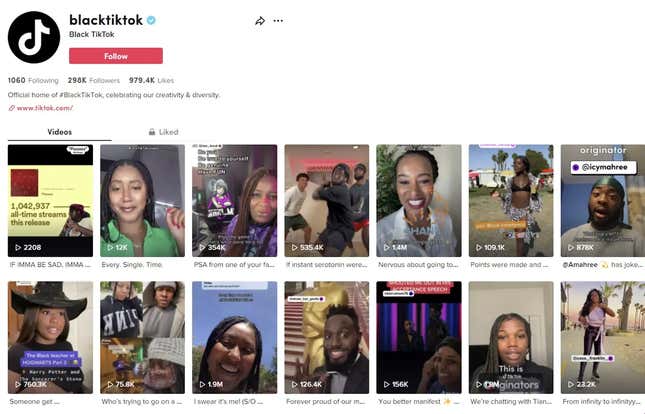The image showcases a TikTok profile titled "Black TikTok," with the TikTok logo prominently displayed in the top left corner. Next to the logo is a blue checkmark indicating verification, followed by the text "Black TikTok" underneath. Below this, a red "Follow" button is featured, accompanied by statistics showing "1060 following," "298k followers," and "979.4k likes."

The profile's bio reads: "Our official home of #BlackTikTok, celebrating our creativity and diversity," with a link to "www.tiktok.com" provided. The interface displays two tabs: "Videos" and "Liked," with the "Videos" tab currently active. The screen showcases a grid of approximately 12 videos arranged in two rows of seven. These videos feature diverse individuals engaging with the camera, including women and men in various attire and settings. Notable thumbnails include a woman wearing a green shirt, a man posing in front of an Oscars-like backdrop, a woman in a black hat, and a video mentioning "over a million all-time streams" in its title. Each thumbnail is accompanied by titles describing the content.